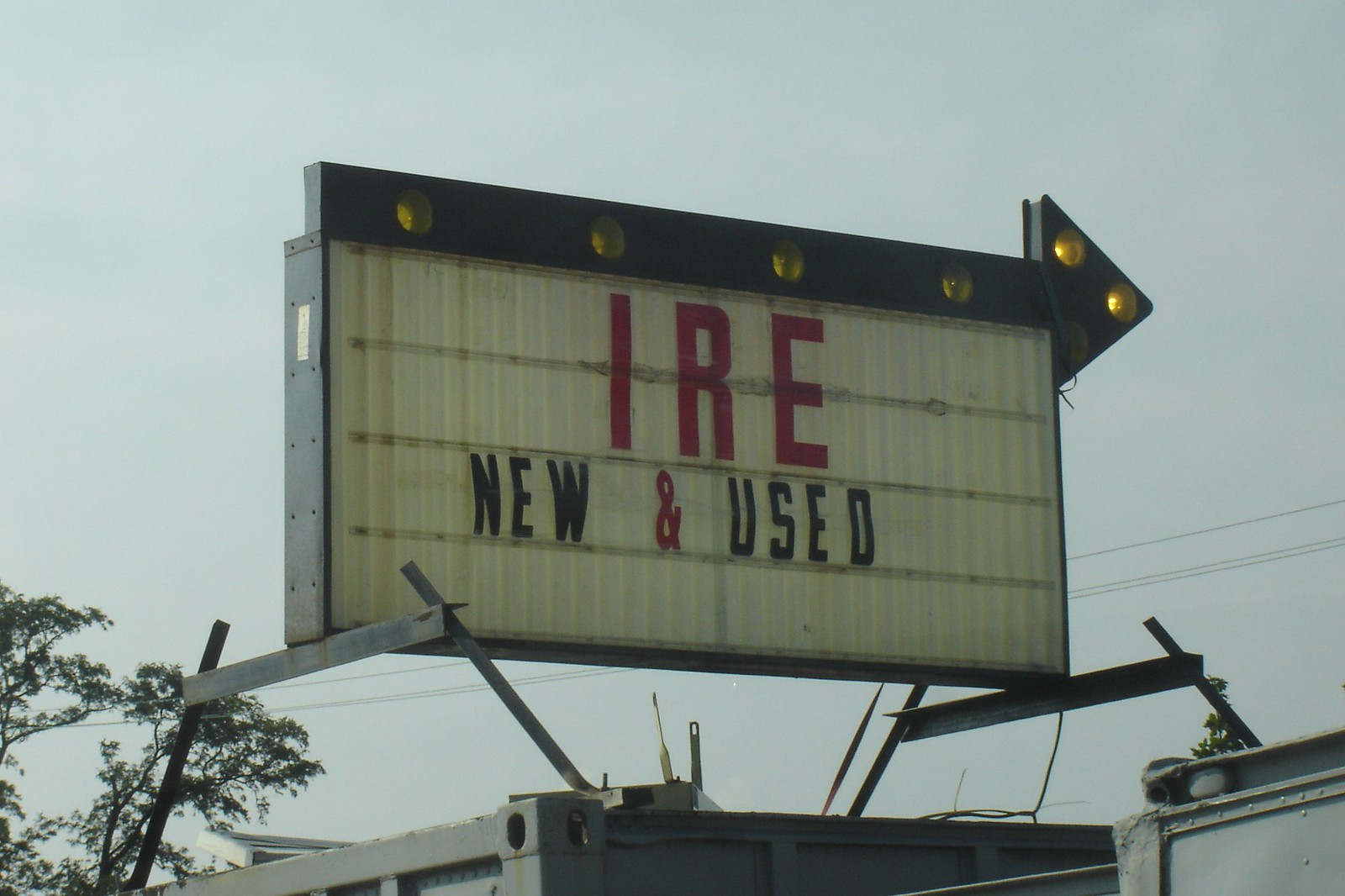The image captures a large, eye-catching portable sign, typically seen in front of businesses, elevated on two gray metal shipping containers. The sign itself has a white background with two horizontal gray stripes across it. The text on the sign is bold and clear: in large red letters, it reads "HIRE," though only "I-R-E" are visible. Below this, in smaller black letters, it says "NEW" and "USED," with an ampersand between them in red. The top of the sign features a black arrow pointing to the right, adorned with yellow or orange light bulbs that outline both the shaft and the triangular head of the arrow, giving it an illuminated appearance. Supporting the sign are sturdy metal beams. The background of the photograph shows a gray, overcast sky, with some power lines, the faint outline of a distant roofline, and the tops of green trees, enhancing the outdoor setting.